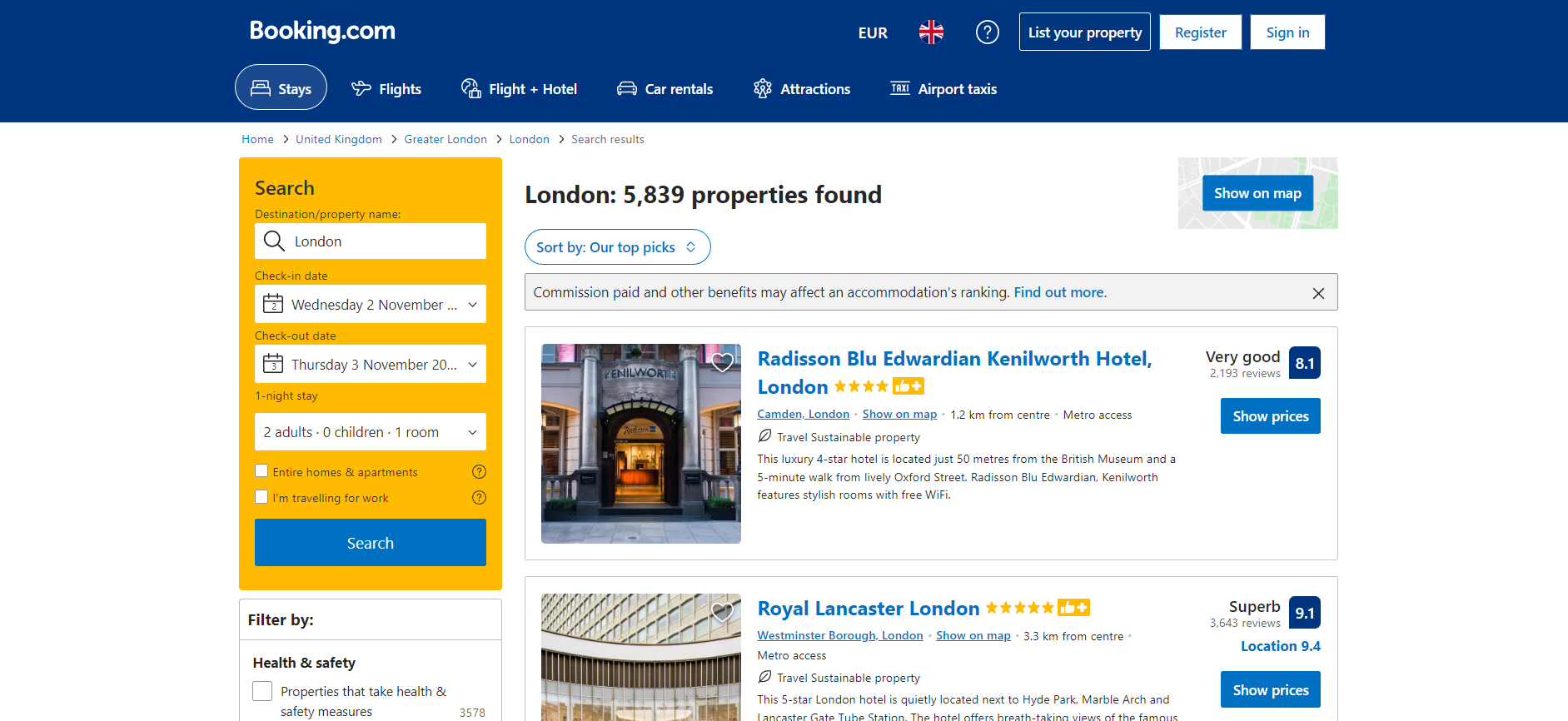The top left corner features the white text "booking.com," highlighting various categories like "Stays," "Flights," "Hotel," "Car Rentals," "Airport Taxis," and "Attractions." Just below these options, to the left, there's a yellow square labeled "Search," containing a search bar where users can input their departure and check-in/check-out dates. 

On the right side of the page, it indicates "London - 5,839 properties found" with a blue button labeled "Show on map" beneath it. 

Displayed prominently is an image of a grand, gray building with tall columns, illuminated from within, suggesting a luxurious setting. This is the Radisson Blu Edwardian Kenilworth Hotel in London, rated four stars with the label "Very Good" beside it.

Adjacent to this, there's another image showing just the ceiling area of another hotel. It's identified as the Royal Lancaster London, boasting a five-star rating and the term "Superb" with a rating score of 9.1 inside a blue box.